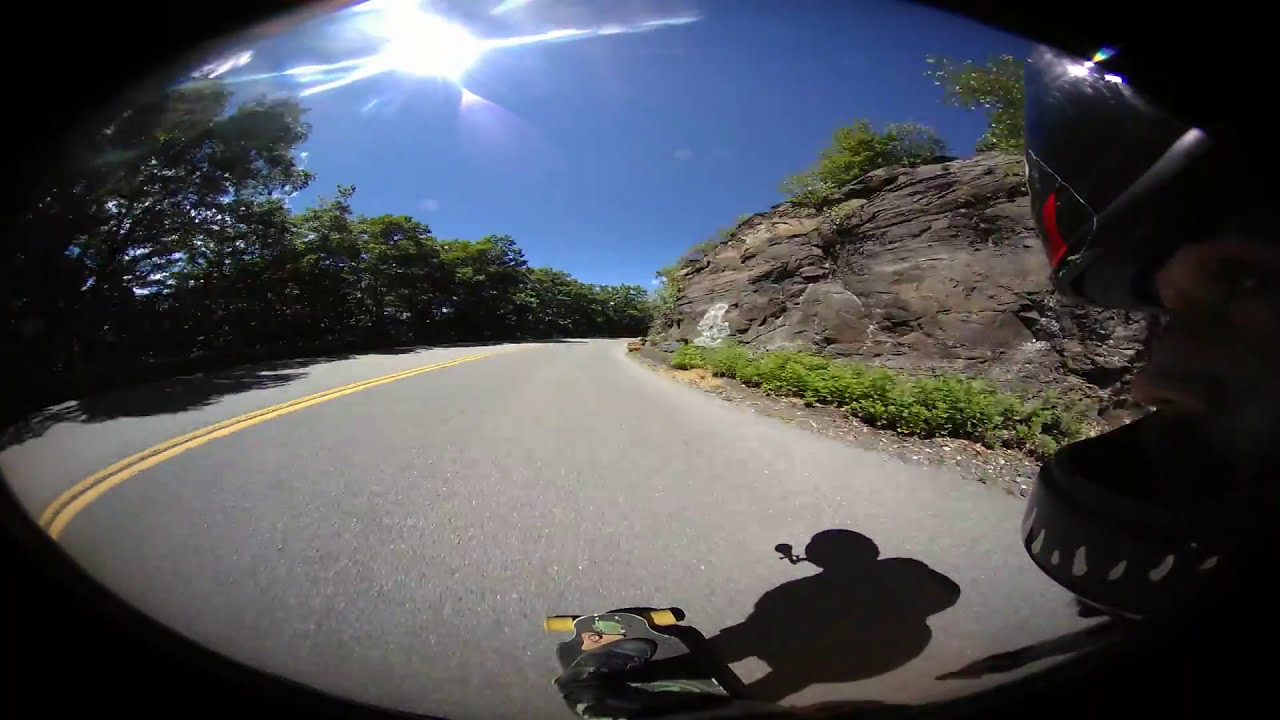The image captures a dynamic scene of a person, equipped with a GoPro mounted on their helmet, riding a longboard down a mountainous road. The fisheye lens effect gives the photograph a curved, circular appearance, enhancing the sense of motion. The rider's feet and the front of the longboard are clearly visible, and their shadow is cast on the sunlit asphalt, which splits into a two-lane road marked by a double yellow line. To the right, the rugged terrain features a rocky cliff adorned with sparse vegetation, while to the left, a dense row of tall trees lines the road. The sky overhead is a clear blue, with a slight sun glare adding to the overall vibrancy of the scene. The outline around the picture suggests it might have been captured by the dash cam of a motorcycle, hinting at a moment of pause in their adventurous ride through the mountains.